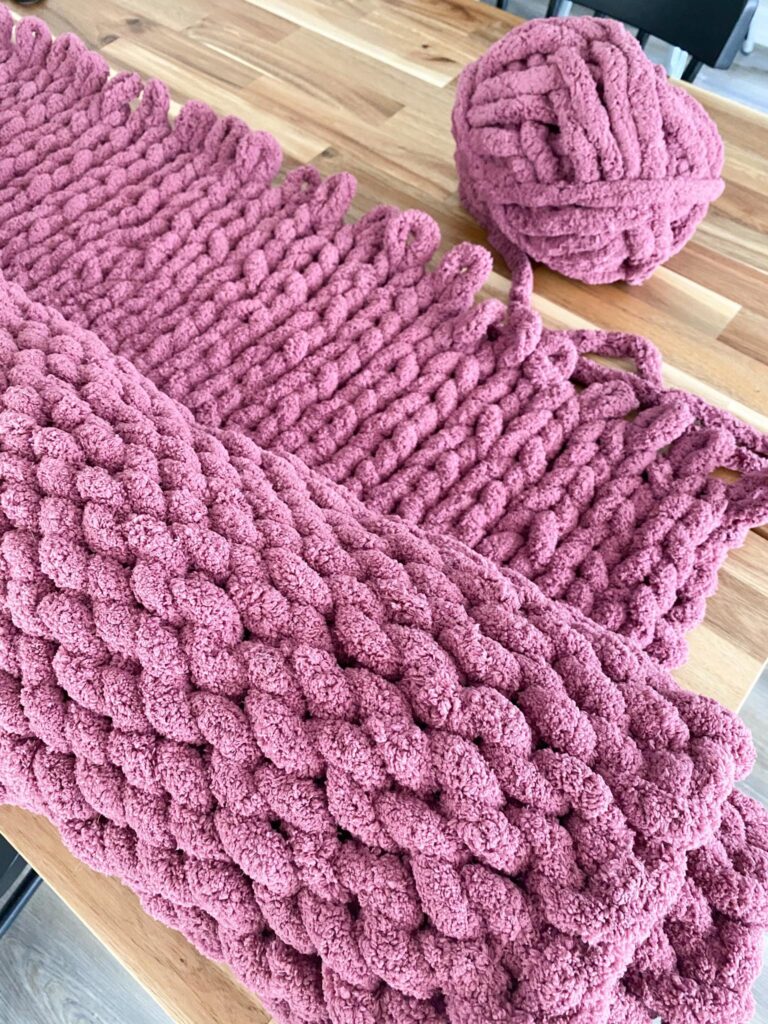This image depicts a nearly finished, rolled-up pink chenille knitted blanket with a chunky texture, exuding a soft and fluffy appearance. The blanket, with its large stitches, rests atop a light wooden tabletop, creating a cozy and inviting scene. Adjacent to the blanket is a ball of the same pink chenille yarn used in its creation, suggesting that the knitting project is almost complete, with only final touches needed. The tabletop, potentially a kitchen or dining table, is complemented by hints of a gray wooden floor beneath and a small visible section of a black chair, adding depth and context to the setting. The photograph is taken at an angle that directs the viewer's eye from the upper right, where the ball of yarn is situated, across the table, emphasizing the continuity of the knitting endeavor.